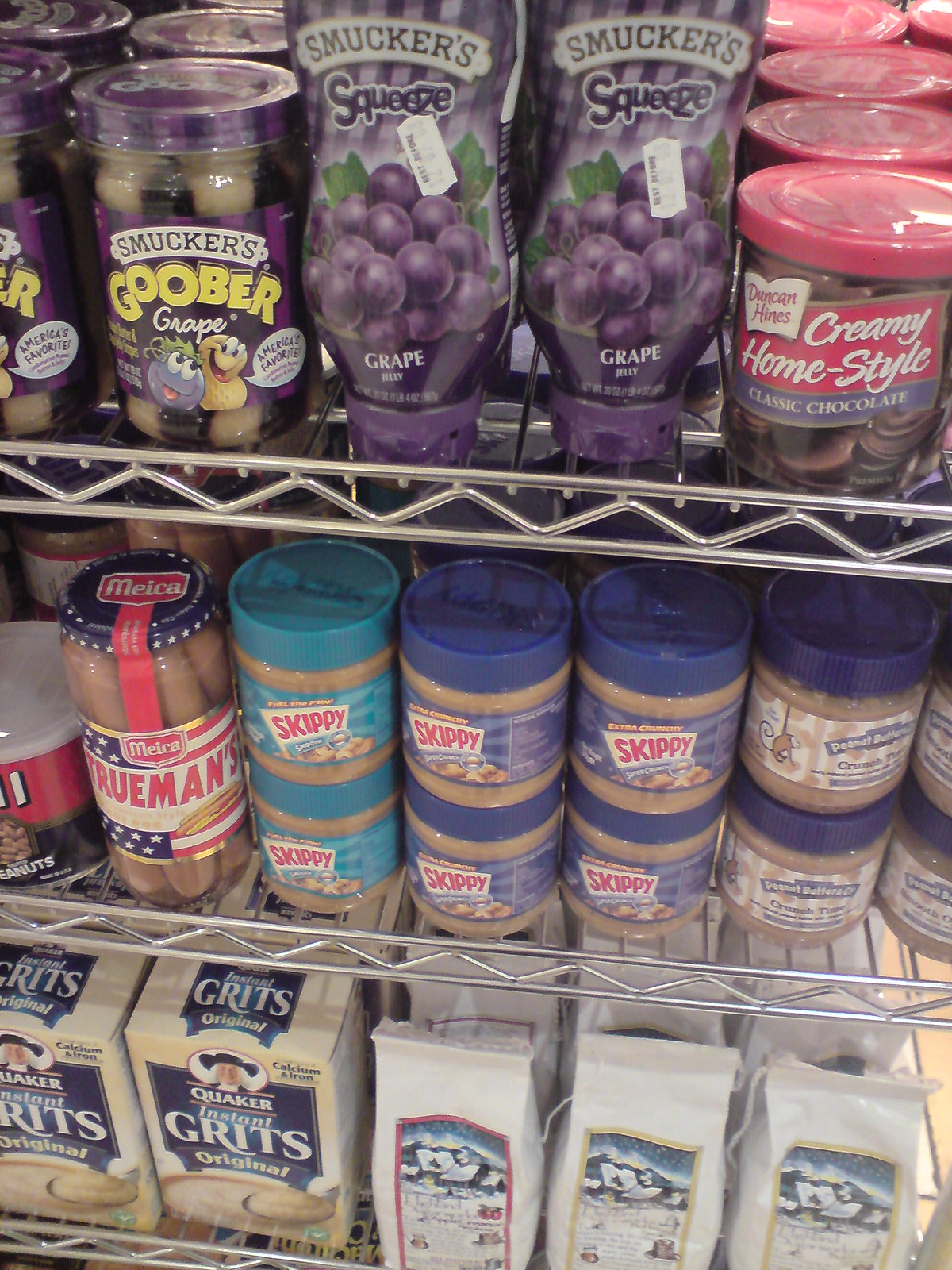This slightly vertical image captures three well-organized shelves in a store. On the top shelf, there are various grape jelly products, including Smucker’s squeeze bottles of classic grape jelly and creamy, home-style chocolate spread housed in a clear container with red caps. The middle shelf features a comprehensive range of Skippy peanut butter jars, which come with turquoise and purple caps, indicating they might range from crunchy to smooth, and potentially even include cookie butter varieties. The bottom shelf displays Quaker Oats grits alongside a mysterious white bag, the contents of which are unclear. The assortment provides a vivid snapshot of the variety of spreads and breakfast foods available in this store.